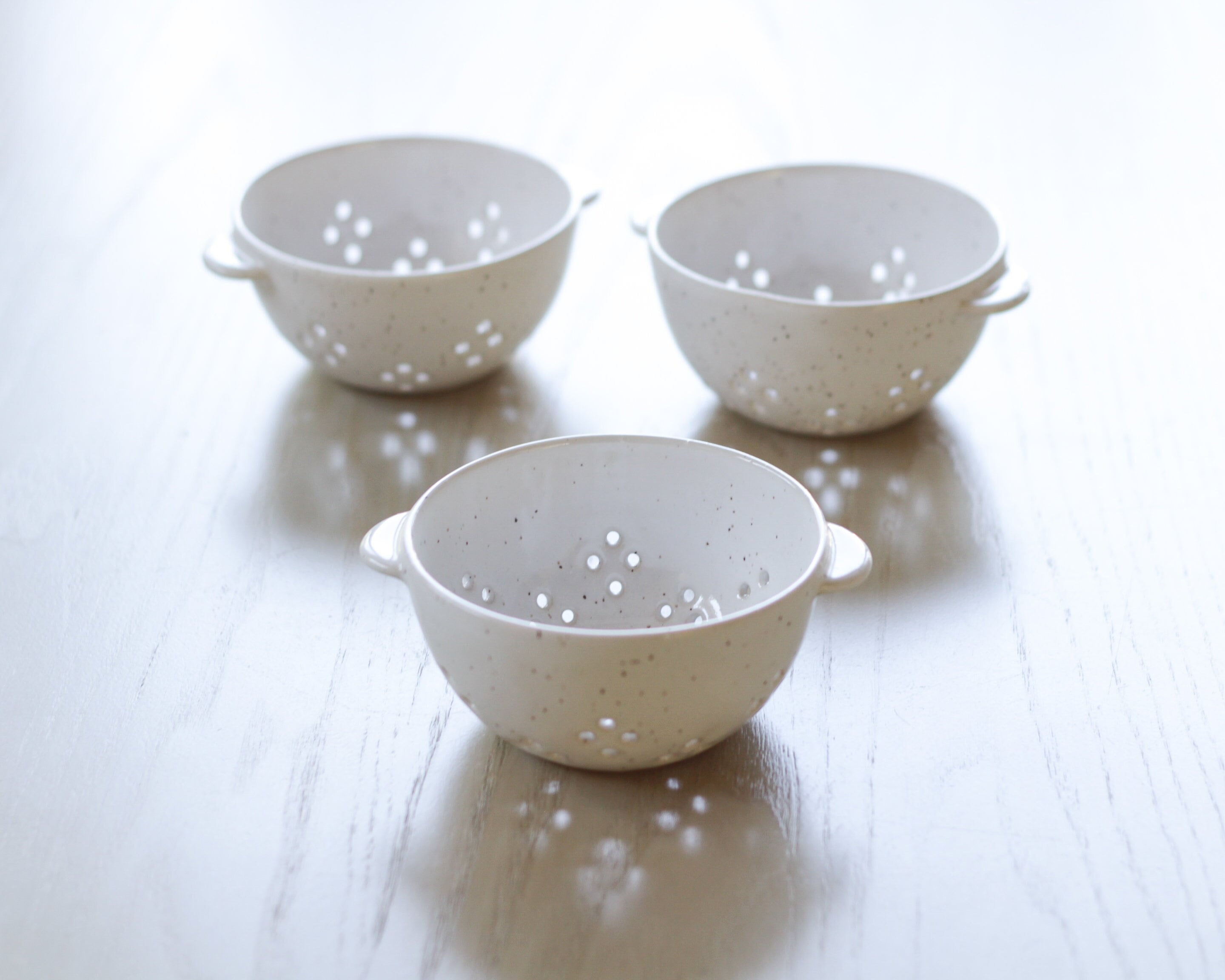The image captures three small, off-white crucibles with dark grey specks, arranged in a triangular formation on a beech wooden table. One crucible is positioned in the foreground while the other two are set slightly behind, with the one on the right slightly forward of the other. Each crucible features small, half-circle handles on the sides and a pattern of diamond-shaped holes, which allow light to pass through and create intricate shadows on the table. The table itself has a prominent wood grain running back to front, and is brightly overexposed at the back, which nearly washes out all details. The crucibles appear empty, with their interiors matching the light cream exterior speckled with black. The bright sunlight streaming through a window casts forward-facing shadows, adding to the elegance of the scene.